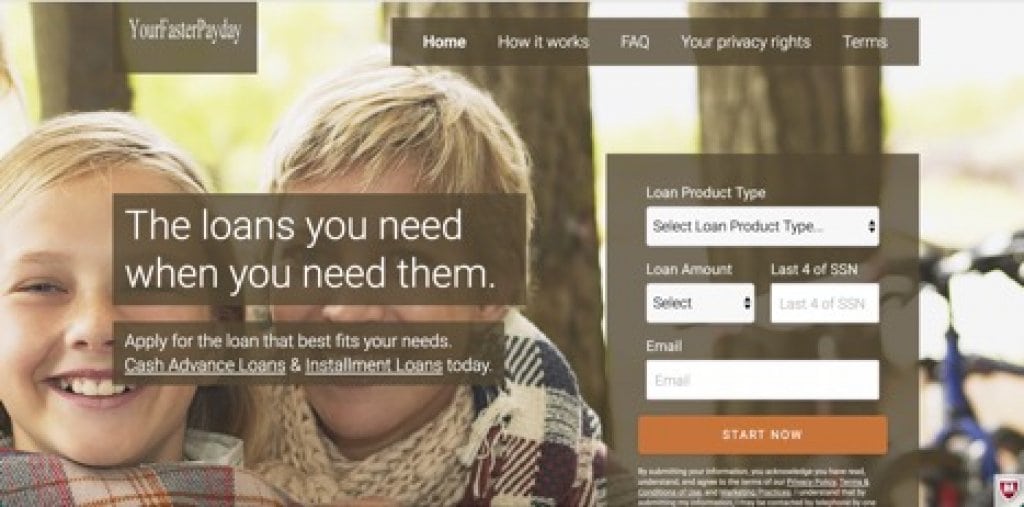This screenshot is from the website "Your Faster Payday." The top navigation bar includes links to "Home," "How It Works," "FAQ," "Your Privacy Rights," and "Terms." The background features an image of two smiling children standing in front of trees with a blue bike leaning against a tree. There may be a second bike, but it's not clearly visible.

Superimposed over the children's faces is the text: "The Loans You Need When You Need Them. Apply for the loan that best fits your needs. Cash advance loans and installment loans today." To the left, there are dropdown menus and input fields labeled "Loan Product Type," "Loan Amount," "Last Four of SSN," and "Email," where users can select loan options and input their information. Below these fields, a large burnt orange button reads "Start Now." At the bottom of this section, there's a line of tiny white text containing terms and conditions, which is too small to read.